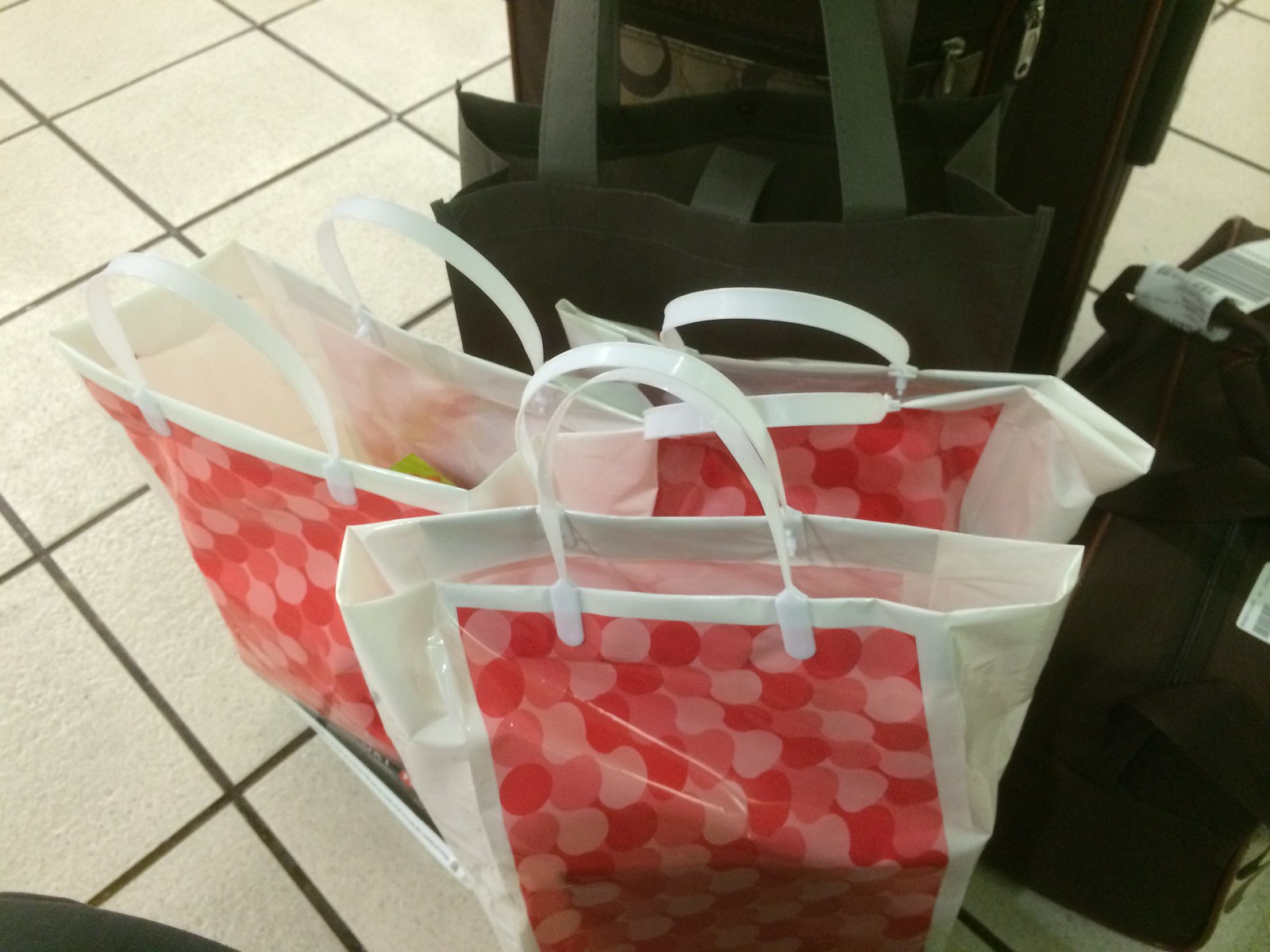The photograph features a tiled floor with large white square tiles separated by dark grout, commonly seen in public places. Sitting prominently in the foreground are three white reusable shopping bags with distinct designs on both the front and back: red circles with a pinkish hue in the middle of each side, and white handles standing upright. The bags are slightly open, revealing some contents, including an object with a hint of green visible in one. Behind these is another canvas-like, possibly black, shopping bag, often used for multiple grocery trips. Further back, partially obscured, is what appears to be a piece of luggage with a baggage claim label and another brown and grey bag featuring the Coach logo. This setup suggests the scene might be at an airport, given the presence of multiple bags, luggage, and the type of flooring. The scene is devoid of people but hints at bustling activity.